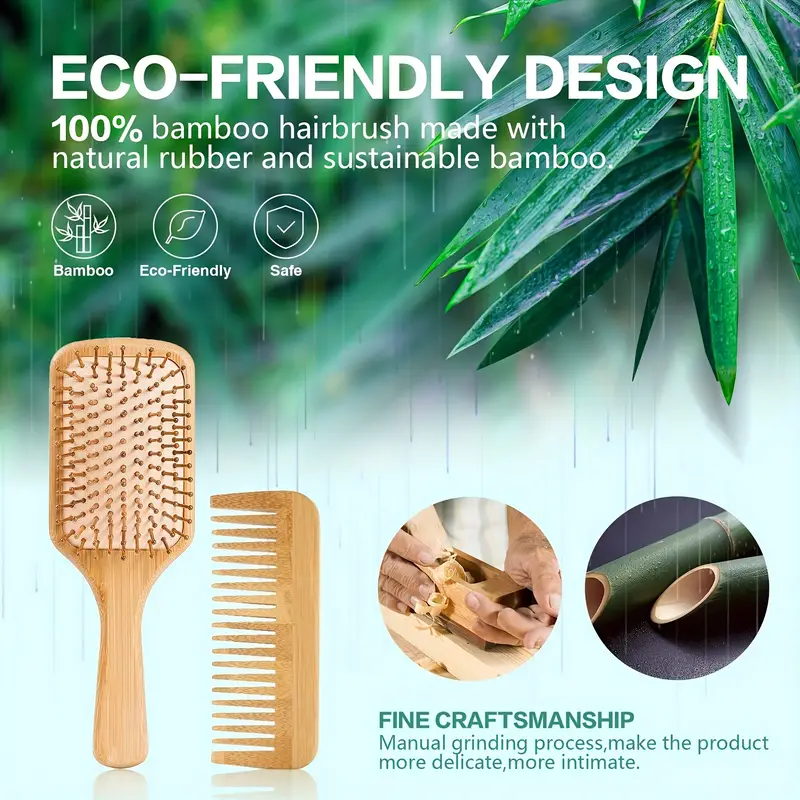The advertisement is slightly vertically rectangular, not quite a square, and features a blurred green background on the left with some out-of-focus plants, and a more defined green plant with long, waxy, rain-covered leaves hanging down from the upper right corner. At the top, large white capital letters proclaim "Eco-Friendly Design." Below this, in smaller print, it states "100% bamboo hairbrush made with natural rubber and sustainable bamboo." Just under this, three round icons are displayed: one labeled "Bamboo" with a bamboo pole and leaves, another labeled "Eco-Friendly" with a leaf icon, and the third labeled "Safe" with a shield and checkmark.

In the bottom-left section of the ad, there is an image of a brown wooden bamboo hairbrush, and next to it, a matching brown wooden comb. Towards the bottom right, two circles feature detailed images: one shows someone's hands manually grinding the bamboo, emphasizing craftsmanship, while the other displays a piece of green bamboo in its natural state. Below these images, green text reads "Fine Craftsmanship," followed by slightly smaller text that says "Manual Grinding Process, Make the Product More Delicate, More Intimate." The overall background of the ad transitions to a light greenish-gray color at the bottom.